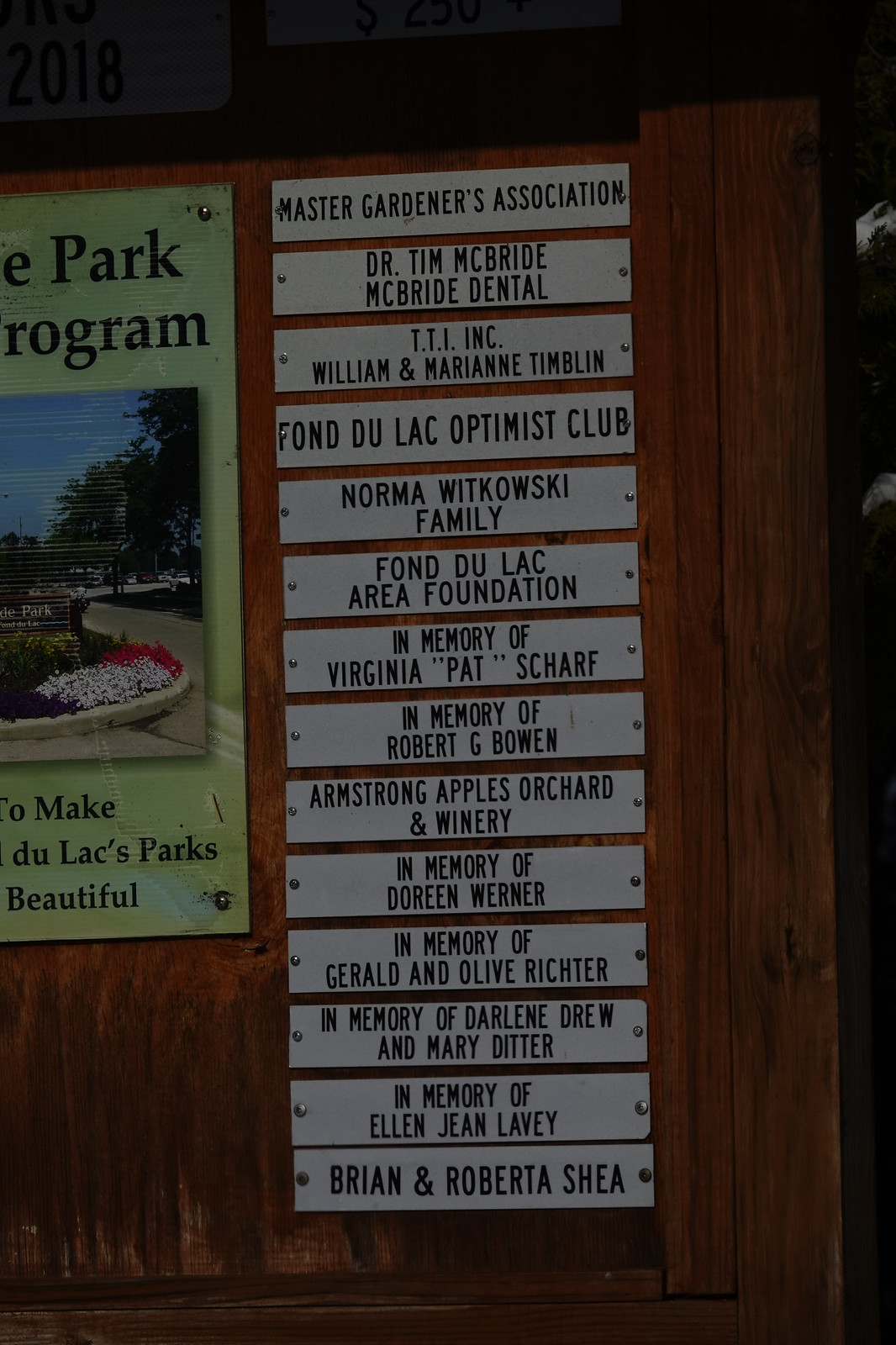In the dimly lit vertical rectangular photograph, a dark wood-paneled wall is adorned with a series of white metal signs in a vertical row. Each sign features black lettering, listing various sponsors and memorials associated with an organization. The signs include names such as the Master Gardeners Association, Dr. Tim McBride McBride Dental, TTI Inc., William and Marianne Timlin, Fond du Lac Optimist Club, Norma Witkowski Family, Fond du Lac Area Foundation, and several memorials including Virginia Pat Scharf, Robert G. Bowen, Doreen Werner, Gerald and Olive Richter, Darlene Drew and Mary Ditter, and Ellen Jean Lavely. The last two entries are Armstrong Apples Orchard and Winery, and Brian and Roberta Shea. Next to these signs, on the left side of the image, a partially visible green poster with black lettering and a photograph in the middle can be seen. The poster includes the word "park" at the top and features a circle with multi-colored flowers in the photograph. This setting is related to the Fond du Lac area, possibly connected to a state park program.